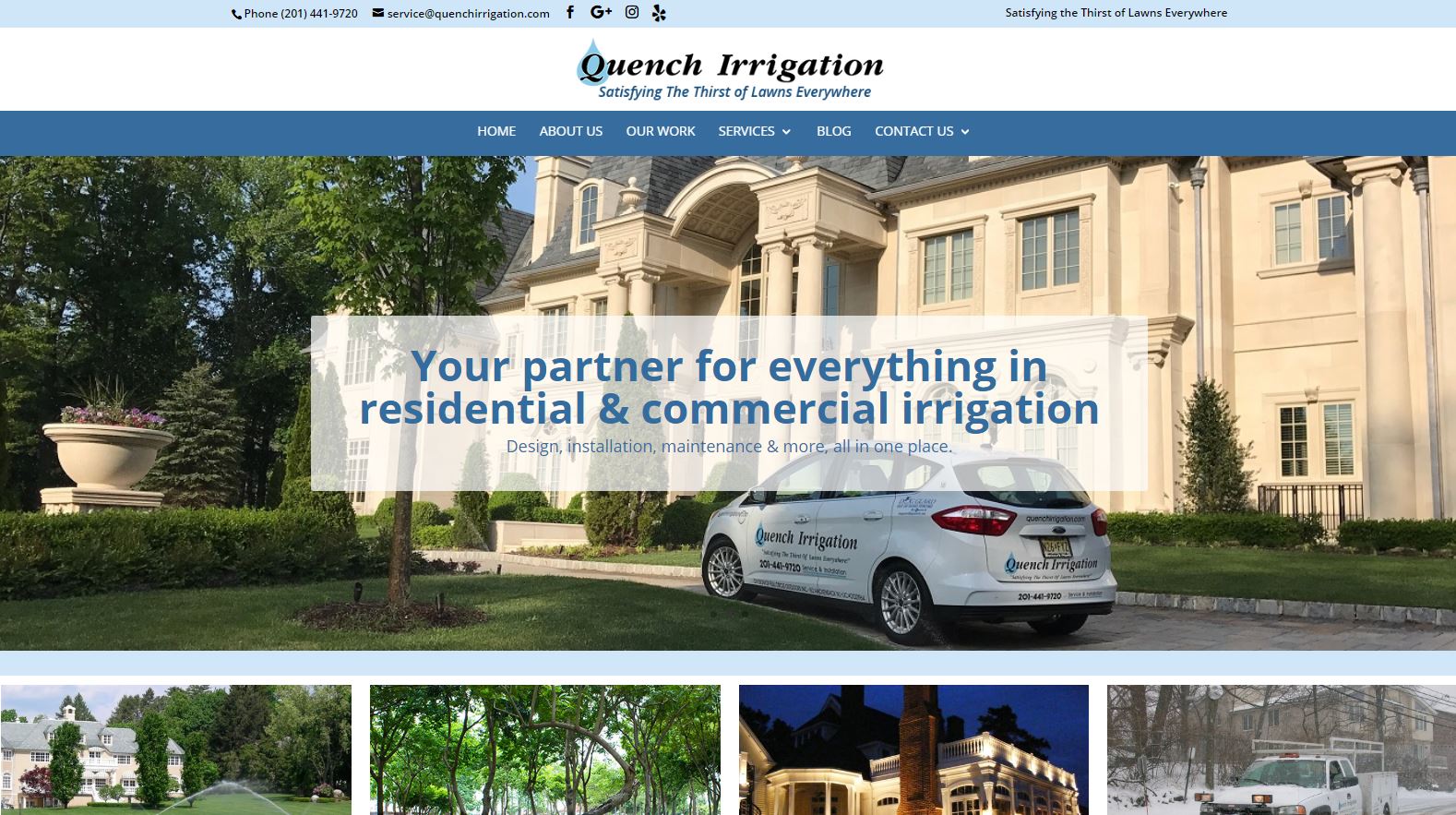This vibrant, detailed website for Quench Irrigation showcases a wealth of information and imagery that highlights their comprehensive irrigation services. At the top, the homepage prominently features a full-color photograph of the Quench Irrigation company car parked in front of an impressive, high-end white stucco mansion, representing the luxurious properties they often service. Below this main image, a series of smaller photographs display other elegant homes and properties, further illustrating the types of prestigious locations that benefit from their expert irrigation solutions.

On the right side of the screen, an image of the company truck parked amidst a snowy landscape underscores their ability to provide irrigation services even in challenging winter conditions. 

The website is rich with content, including detailed sections about Quench Irrigation’s services, company information, and blog updates. Contact information is readily accessible, listing their phone number and email address, along with links to their social media profiles on Facebook, Google Plus, and Instagram. The site proudly touts their slogan, "Your partner for everything in residential and commercial irrigation," highlighting their expertise in both sectors.